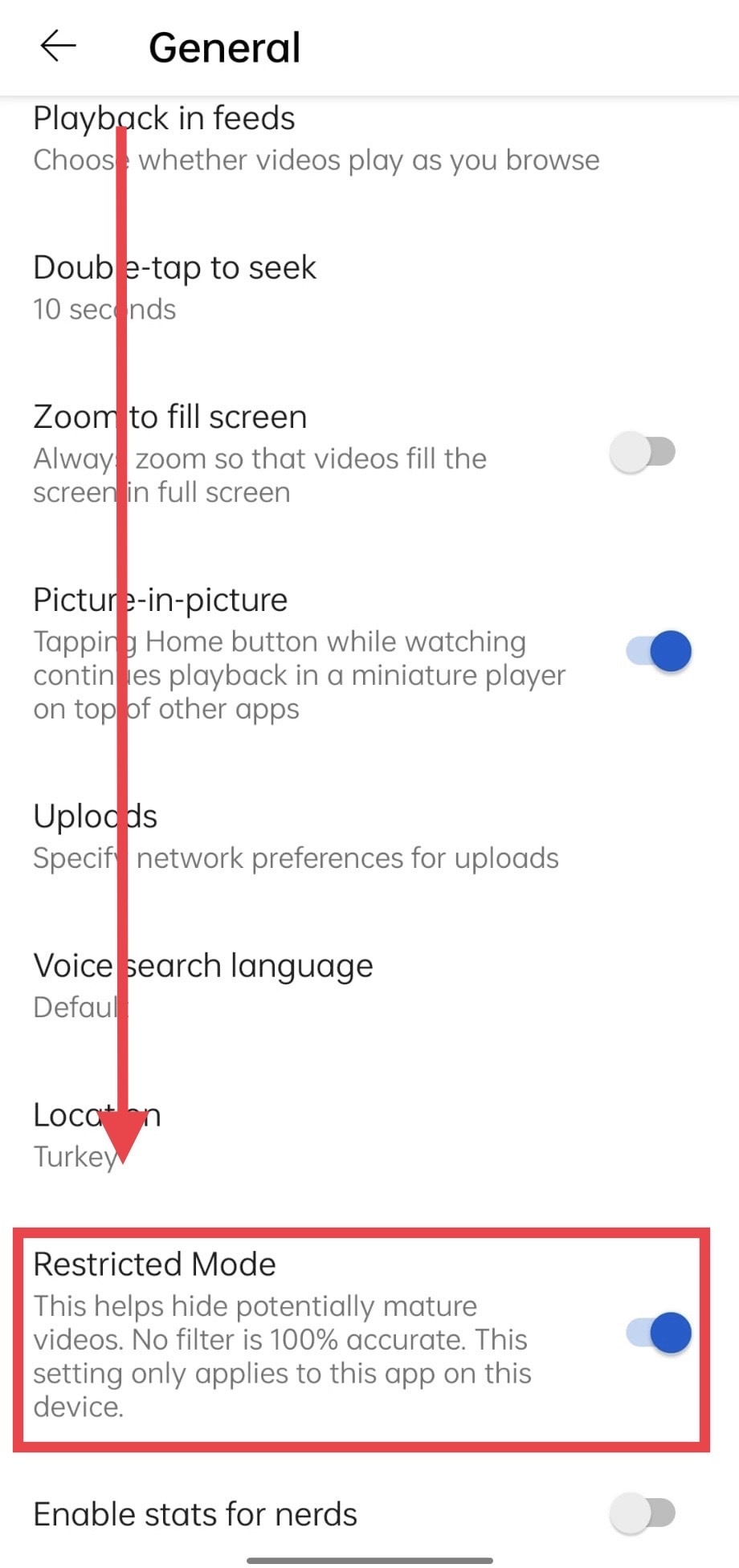The image depicts a smartphone screen displaying a website with various settings under a section titled "General." The screen has a black header labeled "General," followed by several options listed sequentially. The first option, "Playback and Feeds," describes choosing whether videos play as you browse. Below that, "Double Tap to Seek" is set to a default of 10 seconds. The "Zoom to Fill Screen" option, which allows videos to always fill the screen, is currently disabled.

Next, the "Picture in Picture" feature, which continues playback in a miniature player when the home button is tapped, is enabled. Following that, "Uploads" indicates network preferences for uploads, while "Voice Search Language" is set to default and "Location" is set to Turkey.

A prominent red arrow, drawn by someone, starts at "Playback" and spans across all listed options, ending at a red rectangle highlighting "Restricted Mode." This mode, designed to hide potentially mature videos, is currently enabled, suggesting someone is pointing out its importance. The last option, "Enable Stats for Nerds," is also visible and currently disabled. The overall visual emphasizes ensuring "Restricted Mode" is set properly.